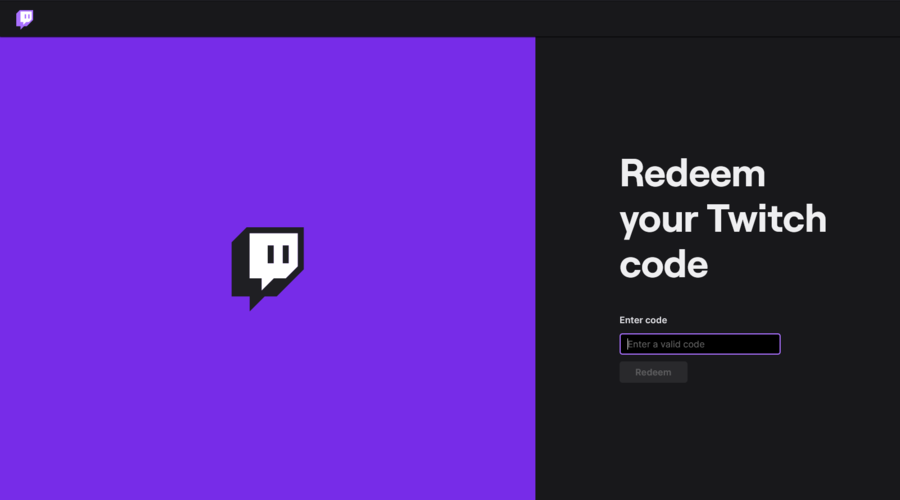The image is a wide rectangular banner, nearly twice as wide as it is tall, characterized by a bold color scheme of black, purple, and white. The layout features a predominantly black background on the right-hand third and a striking purple background on the left-hand two-thirds, separated by a black strip running along the top one-tenth of the entire image.

On the right side, against the black background, there is text in three distinct white lines: "Redeem," "Your Twitch," and "Code," with the initial 'R' in "Redeem" and 'T' in "Twitch" capitalized. Below this text, there is a black, rectangular box outlined in purple, which contains a purple cursor and is labeled "Enter Code" in small white letters above it. Further down, there appears to be a gray button, presumably labeled "Redeem," though the clarity of the word is uncertain.

Dominating the left-hand side of the image, the purple section is interrupted only at the top by the black stripe. Centrally positioned within the purple background is a stylized black-and-white speech bubble icon, shaped like a square with two vertical dashes inside, suggesting conversation or input. This icon is also repeated in the upper left corner within the black top band, rendered in purple and white.

Overall, the composition balances between the dual color blocks, accented with text and interactive elements, creating a visually cohesive and structured layout.